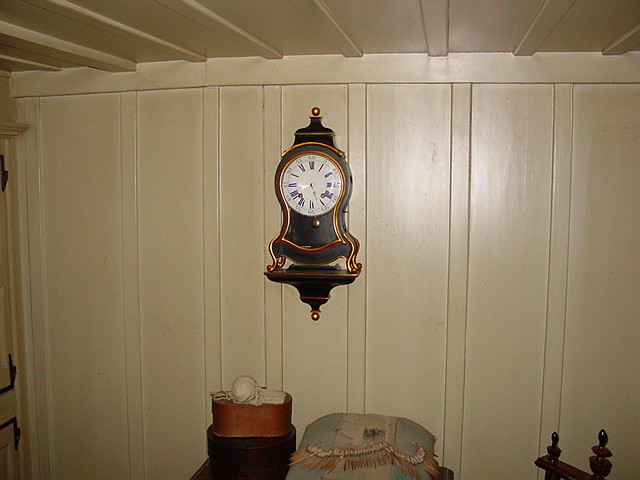The image depicts an ornate clock mounted high on a uniquely paneled wall. The wall and ceiling are painted a beige color, with a distinctive surface created by overlaying wood pieces horizontally and vertically to give it depth and texture before painting. The clock, which appears to date from the early 1900s, features a circular white face with Roman numerals, though the hands are not clearly visible due to the distance. The clock itself is predominantly black with intricate details: it rests on small, gold legs and has a body reminiscent of a little black tummy, complete with a skirt-like design at the bottom. Above the clock face, there's a decorative element resembling a tiny hat with a gold knob on top. The entire clock structure sits on a small platform, adorned with an additional gold knob at the bottom. Below the clock on the floor, there is a pillow and a box containing a circular object.